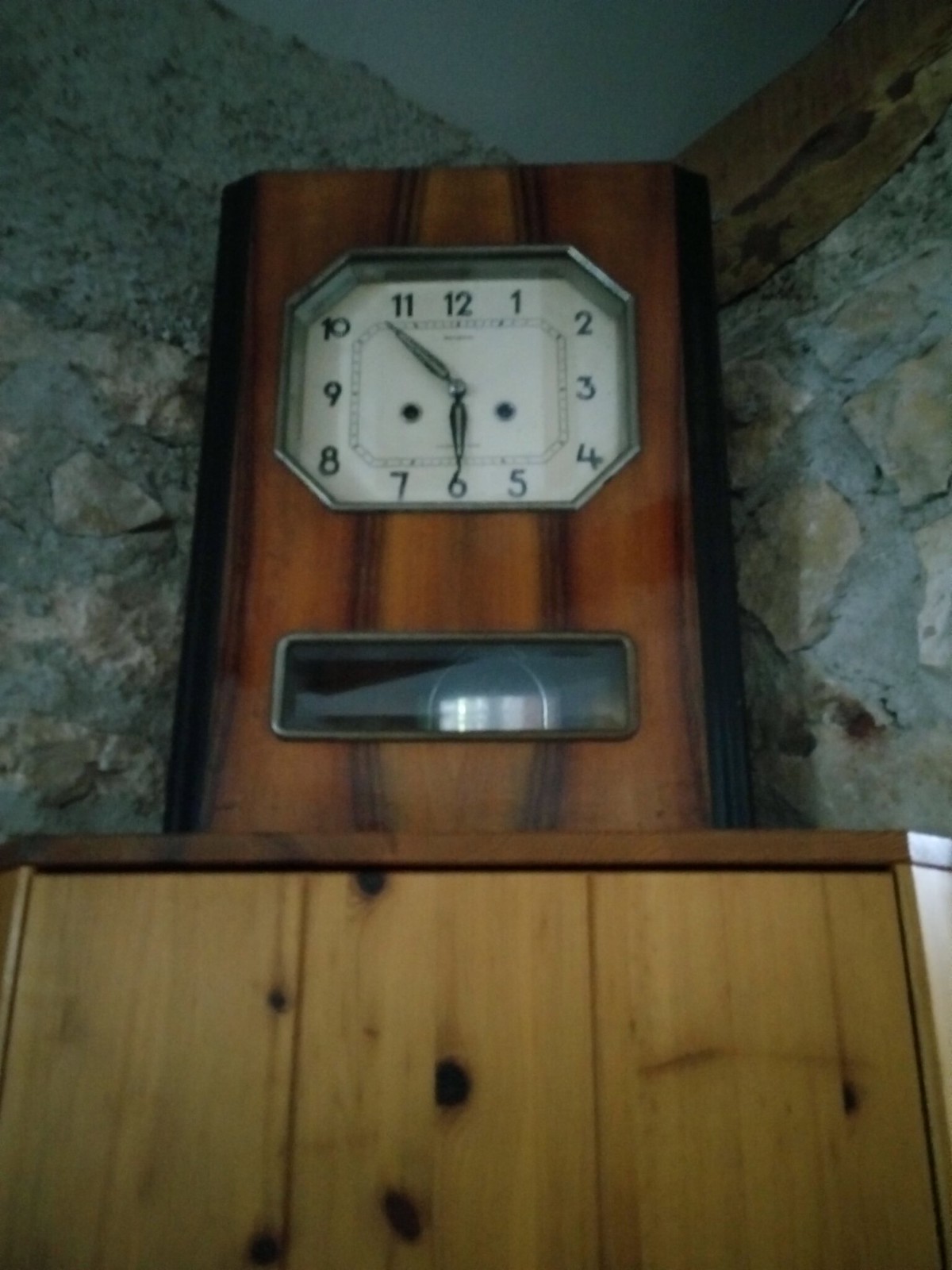This detailed image captures a tall, rectangular wooden clock positioned on top of a light brown wooden cabinet with a slightly darker top. The clock is framed by black vertical borders along its left and right edges, and its body showcases a rich, dark brown wood grain. The clock features an octagonal face with a silver border, displaying black numbers from 1 to 12. The hour and minute hands are black with a hollow design, and they point to 5:53. Below the clock face, there's an inset rectangular section bordered in bronze with clear glass, revealing a silver pendulum inside. The setting is indoors, where the clock and cabinet are situated in the corner formed by two stone walls with visible gray grout between the white-ish stones. The atmospheric stone and mortar add a rustic charm to the scene, which is further complemented by the graceful details of the clock.